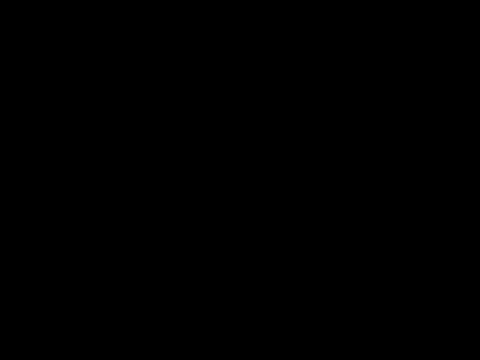The image is a completely black and dark rectangle, devoid of any distinguishable elements or details. There are no objects, no text, and no indication of whether the setting is indoors or outdoors. The only visible feature is an unbroken expanse of black pixels. There are no hints of light or color variations, making it impossible to discern any contextual information. The entire image is uniformly black, giving an impression of either a pitch-black environment or a potential error in the image capture.